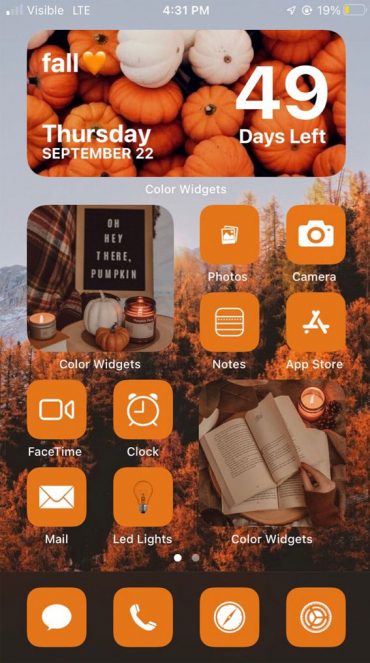The image depicts a screen on a cell phone featuring a fall-themed wallpaper. In the top left corner, the screen displays connectivity bars with the label "Visible LTE," the current time as 4:31 p.m., and the battery level at 19%, indicated in yellow, suggesting it's almost depleted. The central part of the screen is dominated by a horizontal rectangle displaying the word "Fall" with an orange heart emoji, against a pumpkin-themed background. Below this, the date is noted as Thursday, September 22, and it mentions "49 days left," potentially referencing a countdown.

Embedded within the wallpaper is an image of a picturesque hillside adorned with autumn-colored trees, their leaves in vibrant oranges and yellows. Overlaying this scenic backdrop is a widget from "Color Widgets," featuring a pegboard in a coffee shop setting with the phrase "Oh hey there, pumpkin."

The app icons on the screen are themed to match the autumn aesthetic, all in orange with white fonts or symbols. The visible app icons include Photos, Camera, Notes, Apple Store, FaceTime, Clock, Mail, LED Light, Phone, Text, Call, Compass, and an unidentified app represented by circles with a 'Y' inside. The overall theme is consistent with the autumnal motif, showcasing a warm and festive celebration of the fall season.